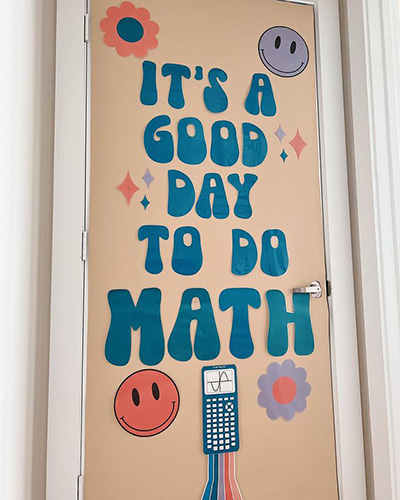This image showcases a decorated doorway, likely from an elementary or middle school participating in a "decorate your door" contest. The background is entirely white, with off-white molding around the door frame. A prominent beige sign covers the entire door, featuring a vibrant and cohesive hippie-inspired design. 

At the top, capitalized blue letters spell out, "It's a good day to do math," reminiscent of the bubbly lettering seen on Grateful Dead or tie-dye shirts. The sign includes an array of colorful elements: an orange flower at the top left, a purple flower at the bottom right, a purple smiley face at the top right, and an orange-red smiley face at the bottom left. Centrally positioned at the bottom is a detailed calculator, possibly a TI-89, colored blue to match the text, with a rainbow gradient extending from its base. 

The consistent color scheme of oranges, purples, reds, and blues ties the entire artistic presentation together, giving it a vibrant, cheerful, and harmonious appearance.